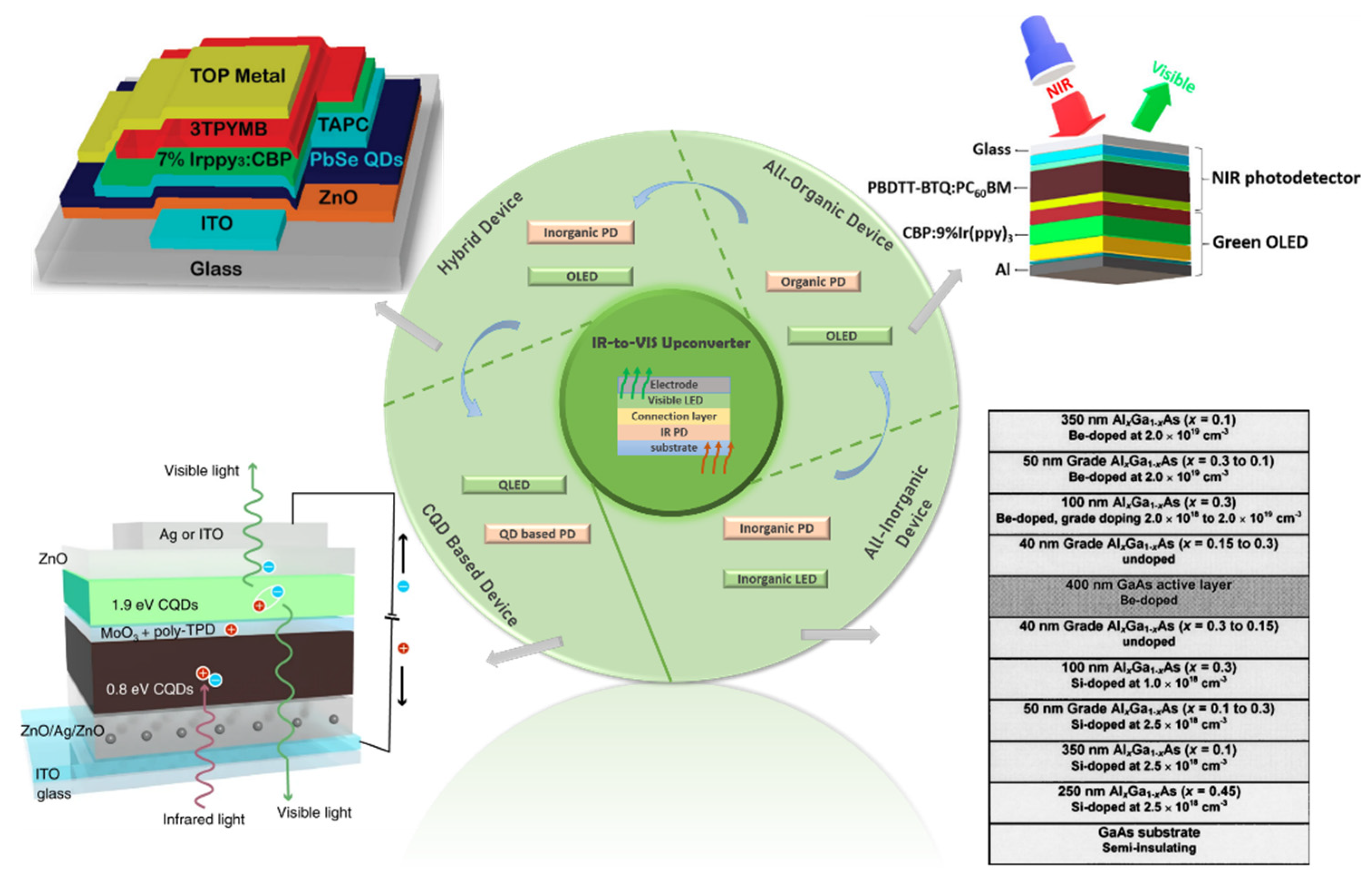This image showcases a detailed, illustrated diagram, likely from a textbook, that appears to depict various types of technological devices. At the center of the diagram, there's a dual-colored green circle, with a dark green inner circle labeled "IR to VIS upconverter," enclosed by a light green outer circle. Surrounding this central circle are four quadrants, each representing different types of devices: "Hybrid Device" (upper left), "All Organic Device" (upper right), "CQD Based Device" (lower left), and "All Inorganic Device" (lower right).

The diagram includes several 3D structural illustrations. In the upper left quadrant, the hybrid device section points to a pyramid-shaped, multi-layered structure with labels like "Glass" at the base and various metals on top. The upper right quadrant features flat, stacked layers of colors, including yellow, red, green, blue, and gray, with labels such as "Top Metal," "3TPYMB," and "TAPC." The lower left quadrant mirrors this pattern, showing another multi-layered formation of glass. The lower right quadrant points to columns filled with scientific texts, equations, and numbers, possibly including measurements like "100 nm."

This complex diagram appears to involve concepts related to infrared and visible light conversion, material science, and perhaps device manufacturing processes, containing numerous scientific notations and equations.